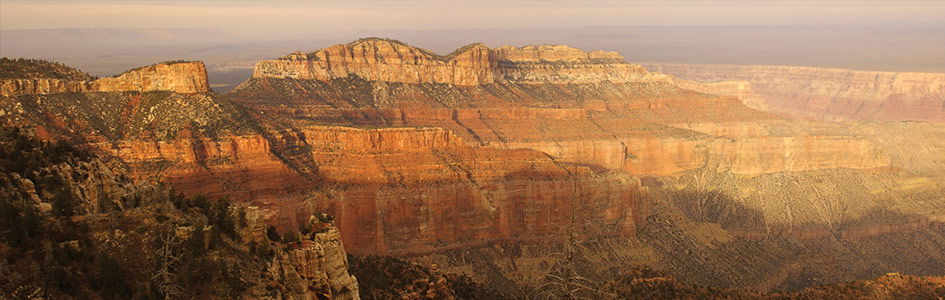This wide, horizontal landscape photo captures a stunning view of the Grand Canyon. The image is framed within a narrow rectangle, showcasing the majestic cliffside from a long distance. Prominent rock formations dominate both the left and right sides of the picture, each displaying a layering of sediment accumulated over millennia. These layers range in color from deep reddish-brown at the bottom to grayish-brown in the middle, capped with lighter tan and white rocks at the top. The middle sections feature patches of foliage and greenery, while the top and bottom sections remain relatively barren. Although taken during daylight, the sky is overcast with a gray hue, casting a softer light that creates slight variations in brightness across the image, making the left side appear somewhat darker than the right. The photo likely captures the scene later in the afternoon, given the muted sunlight.